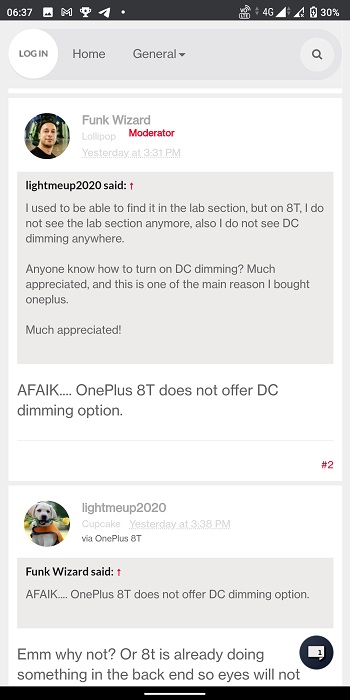In this smartphone screenshot, the interface presents three tabs on the top-left corner: "Login," "Home," and "General". The "Login" tab is highlighted in white, indicating the current selection, while "Home" and "General" are greyed out. On the top-right corner, there's a search icon. 

The main content of the page is a discussion involving two users, "Light Me Up 2020" and "Funky Wizard." Prominently, at the top of the discussion, in black text, is the username "Funky Wizard," followed by the word "Lollipop" and the term "Moderate," which is written in red. This indicates the user rank or role. The timestamp for the post is "Yesterday, 3:31 PM." 

"Light Me Up 2020" has a profile picture on the right side of the post, showing a person wearing a black cap and a black T-shirt. Underneath, their post reads: "I used to be able to find it in the left section, but on the 8T, I do not see the left section anymore. Also, I do not see DC Dimming anywhere. Anyone who knows how to turn on DC Dimming, much appreciated. This is one of the main reasons I bought OnePlus. Much appreciated." 

Funky Wizard replied to this post stating that the "OnePlus 8T does not offer DC Dimming option," addressing "Light Me Up 2020," whose nickname on this service appears as "Cupcake." 

"Light Me Up 2020" has another profile picture showing a white dog holding yellow and green flowers in its mouth while wearing an orange vest. They responded to Funky Wizard at "Yesterday, 3:38 PM," with: "Why not, or the 8T is already doing something in the background, and so eyes will not..." The post abruptly ends there, leaving the reader curious about the rest of the message. The user's device is identified as OnePlus 8T.